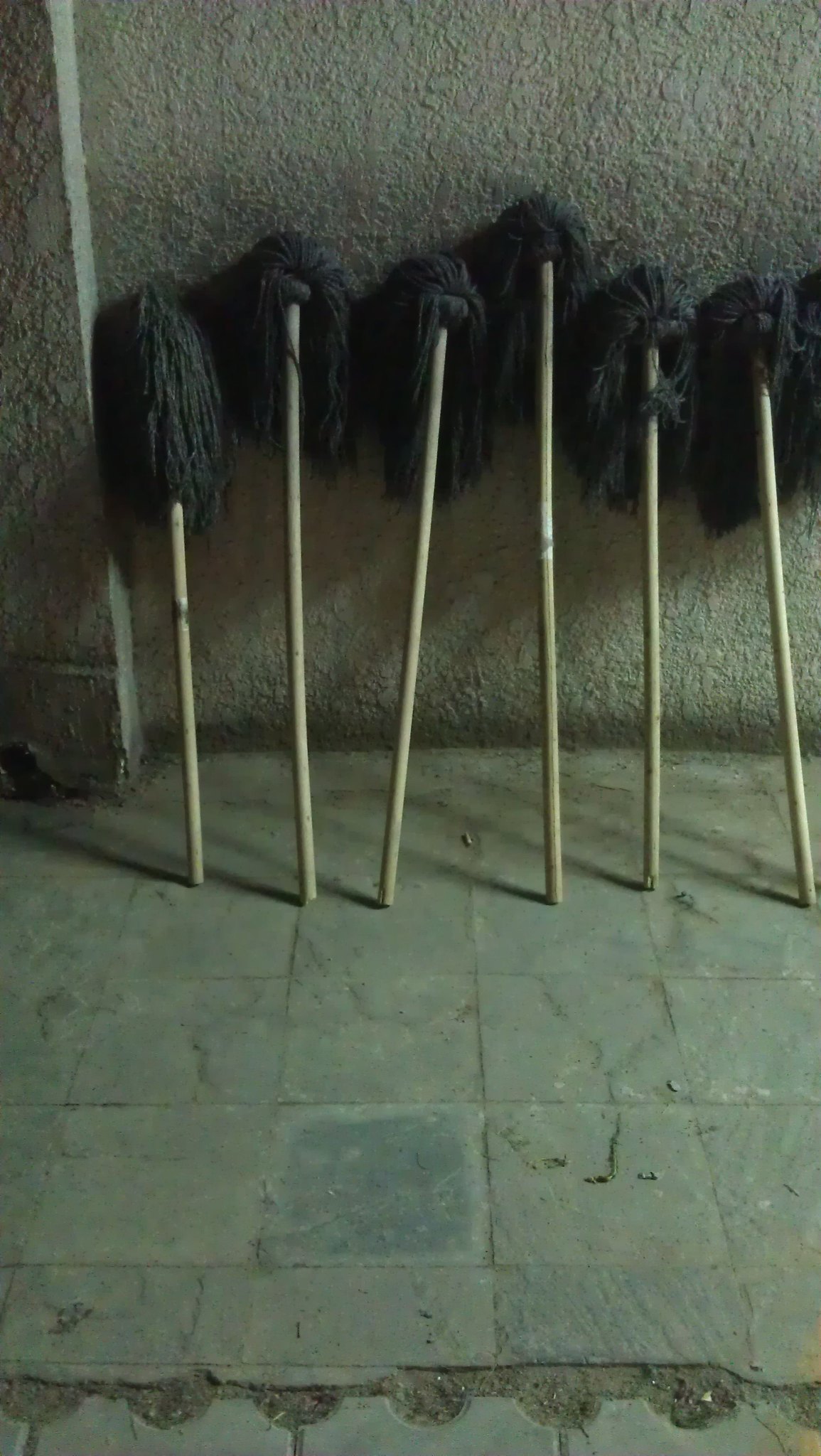In this image, there are six mops with dark gray to black mop heads and light tan wooden handles, all leaning against a rough, textured stone wall, which has a section that juts out slightly. The ground consists of worn, grayish tiles, with some tiles chipped or coated in dirt, revealing patches of dirt between them and contributing to a somewhat neglected outdoor environment. The scene is further marked by a small mound of dirt against the wall, adding to the overall impression of an area frequently exposed to the elements and usage. The mops, resembling disheveled wigs atop sticks, provide a stark contrast against the austere backdrop of the concrete stucco wall and weathered flooring.